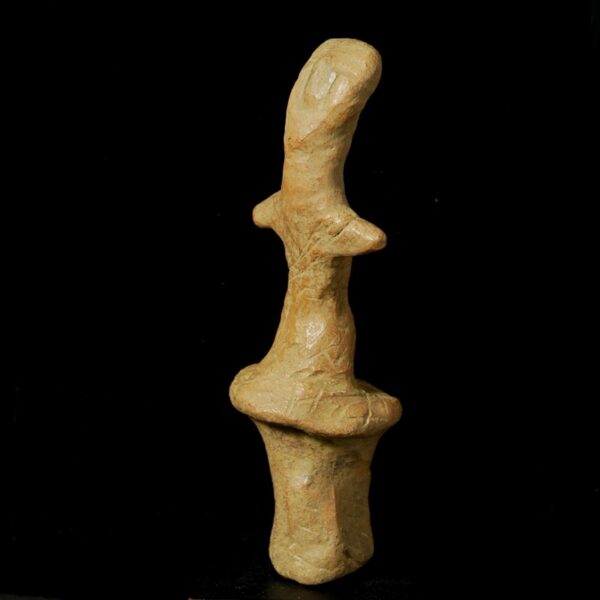In the center of the image, set against a deep, solid black background, stands a narrow, vertical artifact that extends from the bottom to the top of the frame. This sculpture, likely displayed in an art or history museum, is predominantly brown with various shades adding depth to its appearance. The base of the artifact is wider, resembling something that could be gripped with a fist, gradually narrowing upwards with two rounded points or "stubby arms" protruding from the midsection. The upper part tapers into a rounded tip, maintaining the narrowness of the middle portion. The artifact's shape evokes the form of a person, with a broader base akin to hips, two small arms, and a rounded head, making it reminiscent of both an ancient relic and a stylized human figure. The sculpture stands in stark contrast against the dark background, highlighting its intricate details.